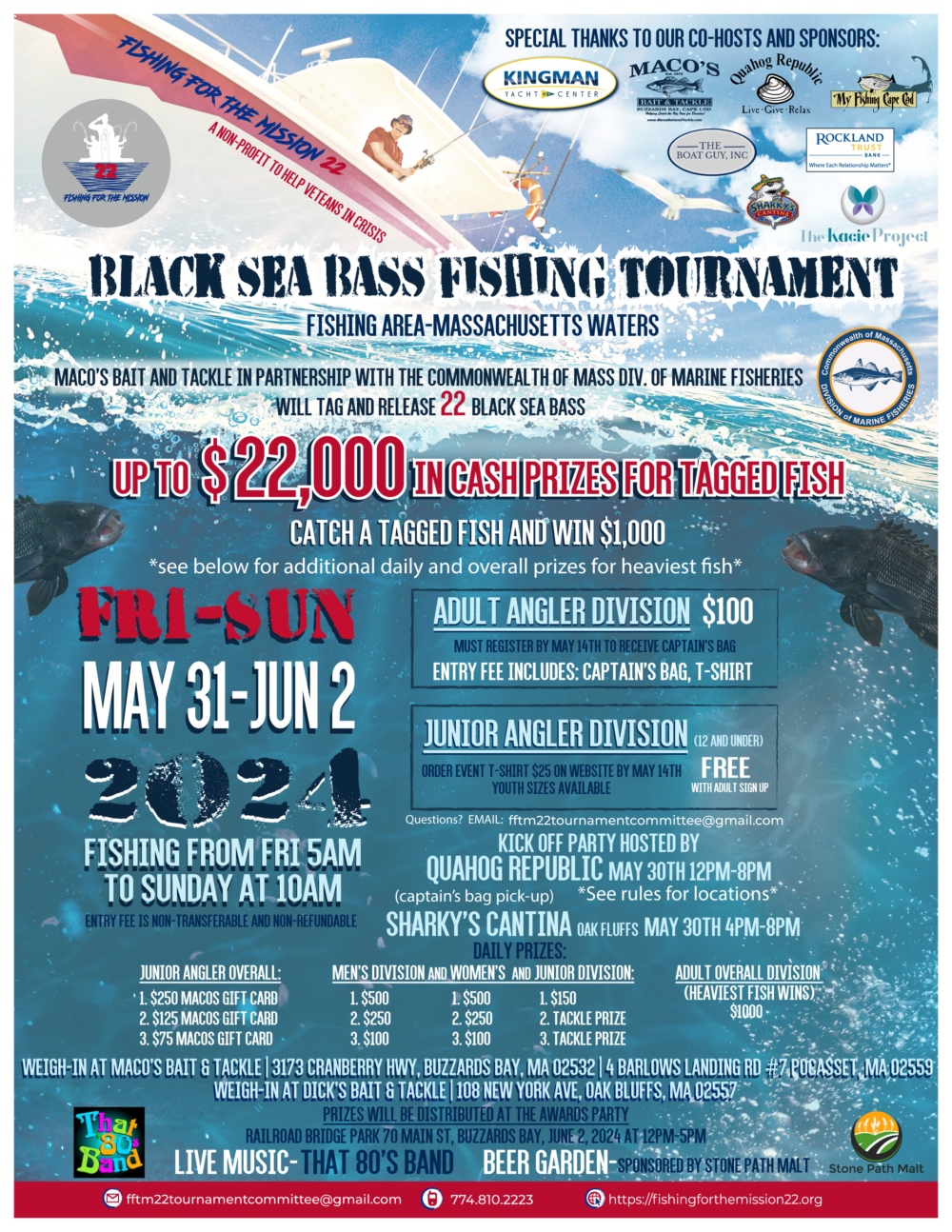The poster for the Black Sea Bass Fishing Tournament is a beautifully designed and detailed promotional image. At the top of the poster, the title "Black Sea Bass Fishing Tournament" is prominently displayed in black stenciled text, with a smaller subtitle "Fishing Area - Massachusetts Waters" below it. On the top left, a white boat with a pink stripe and blue text stating "Fishing for the Mission 22" is depicted, highlighting the nonprofit's mission to help victims in crisis. A man, equipped with fishing gear and wearing a hat, stands on the boat actively fishing. 

In the top right corner, numerous sponsor logos are arranged under the heading "Special thanks to our co-hosts and sponsors," including notable names such as Kingman, Mackoast, and Rockland Trust. The middle of the poster announces bold event details and prizes, stating "Up to $22,000 in cash prizes for the tagged fish" and giving the event dates as "Friday to Sunday, May 31st to June 2nd, 2024" in vivid red text. Additionally, it's highlighted that MAKO's bait and tackle, with the Commonwealth of Massachusetts Division of Marine Fisheries, will tag and release 22 black seabass, each worth $1,000 if caught.

The lower section of the poster provides logistical information, noting that fishing will occur from Friday at 5 AM to Sunday at 10 AM. The entry fee for the adult angler division is $100, which includes a captain's bag and a t-shirt, while the junior angler division (12 and under) is free with an adult sign-up. There's also a note that event t-shirts can be pre-ordered for $25 on the website by May 14th, with various sizes available.

The overall style of the poster combines photographic representation with graphic design, featuring an underwater view of fish and a striking visual of the boat above, creating a dynamic and engaging promotional piece.